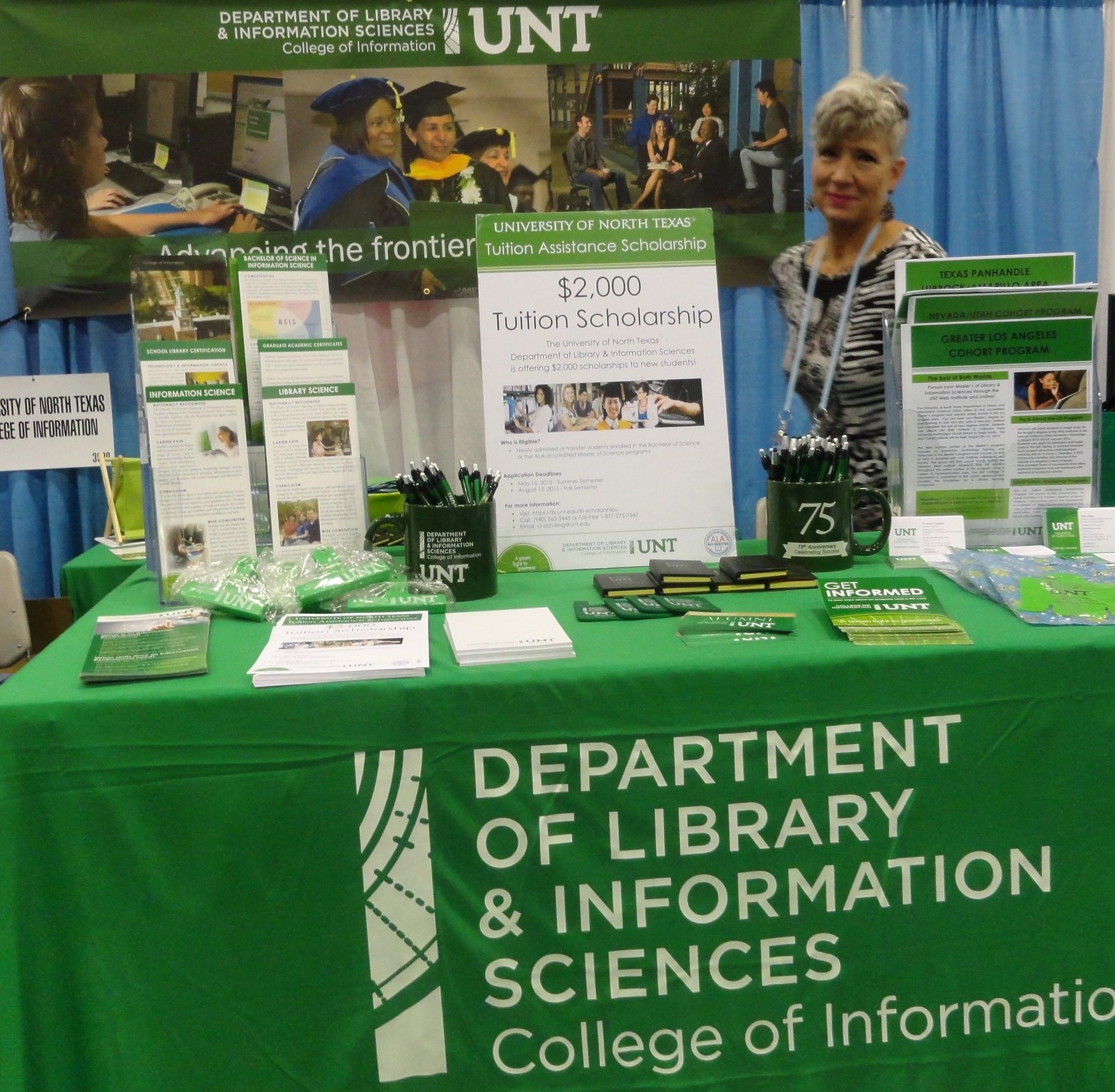This photograph depicts a booth at a conference or convention, prominently featuring the Department of Library and Information Sciences from the College of Information at the University of North Texas (UNT). The booth, adorned with a green tablecloth and white lettering, showcases the university's colors. Behind the table stands a woman with short gray hair, smiling at the camera. She wears a black and white zebra-striped dress and a blue lanyard with a badge around her neck.

The booth's backdrop includes a detailed banner with the department's name, the UNT logo, and photographs of students engaged in various academic activities—working at a computer, interacting in class, and during graduation. The table is covered with numerous informational brochures, pamphlets, and flyers about the department and its offerings. Various giveaways are neatly arranged, including pens in coffee cups, notebooks, sticky notepads, chip clips, koozies, and items in small bags. A prominent sign in the center of the table announces a $2,000 tuition scholarship for prospective students. Blue curtains form the background, completing the booth's professional and welcoming appearance.